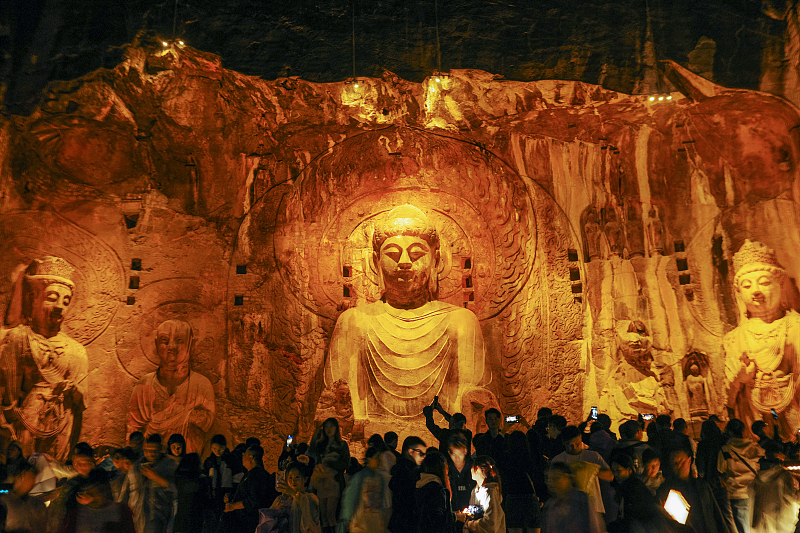The photograph captures a captivating scene within a cave, heavily adorned with Buddhist statuary. Centered prominently is a large statue of Buddha, seemingly carved directly into the rough, sandstone-like rock wall that envelops this sacred space. The Buddha statue exudes a golden hue under warm, focused lighting, which also highlights its intricate halo-like carvings around it. Flanking the central figure are two smaller monk statues on either side, while further to the left and right stand additional identical monk statues, each seemingly armored and donning a distinct hat.

The cave itself, with its dark, rough, and curved ceiling, almost cloaks the entire scene in a mystical ambiance, enhanced by the night time setting. The low, warm lighting adds to this enchanting atmosphere, casting the sculptures in a serene glow while keeping the background shadowy. Below these grand statues, a sizable tourist group is gathered, many dressed in long-sleeved coats and jeans, eagerly capturing the moment with their smartphones. Their illuminated screens and flashes create a subtle contrast against the otherwise dimly lit environment, emphasizing the reverence and awe inspired by these monumental Buddhist carvings.